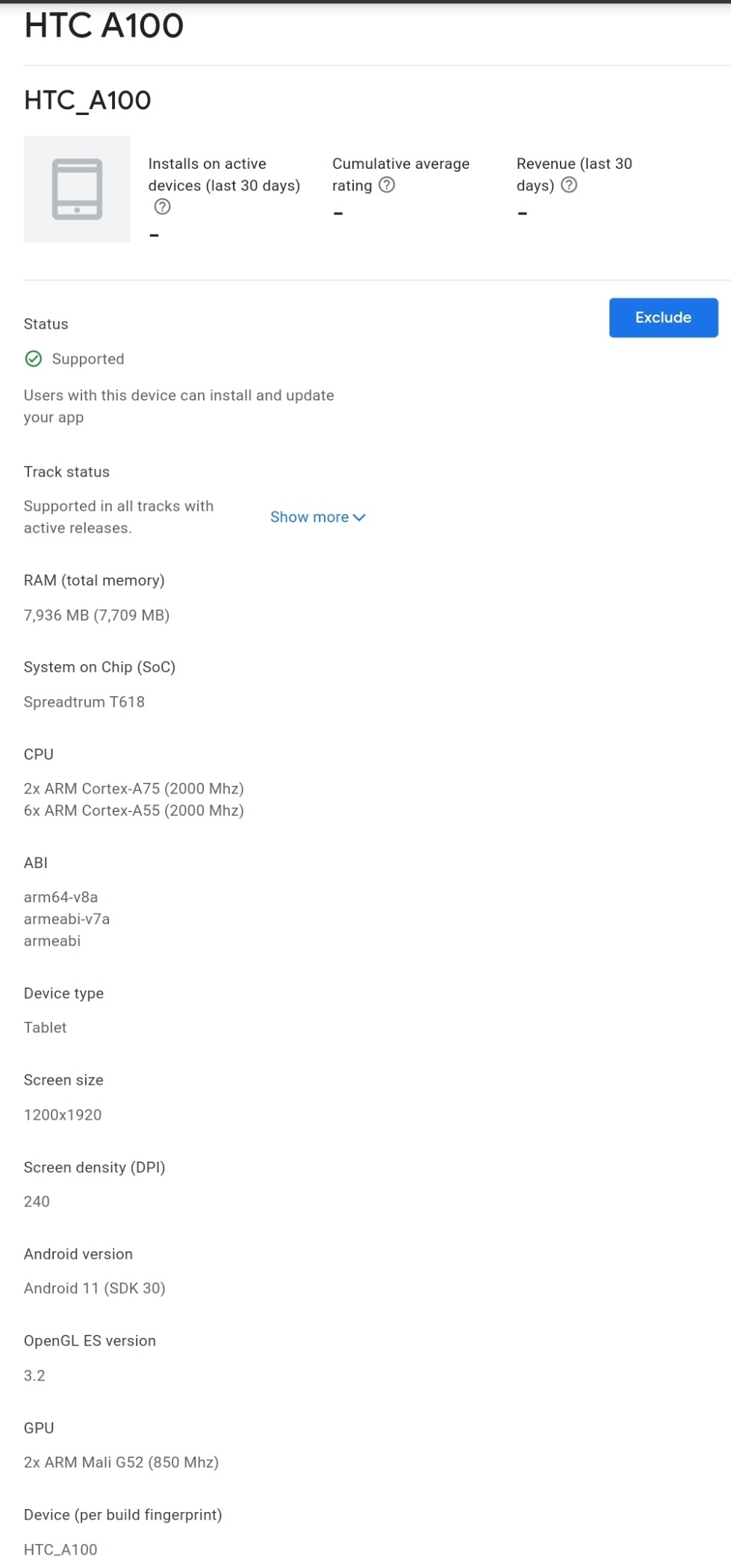The image showcases a detailed dashboard for a device referred to as HCCA 100. The central theme is presented in bold black letters against a white background, featuring the title "HCCA 100." Below this heading, there is an illustration resembling a tab on a smartphone, accompanied by several metrics and statistics. The metrics include recent installations of active devices over the past 30 days, cumulative average ratings, and revenue figures for the same period. 

A horizontal line divides the section, beneath which there is a blue button labeled "Exclude" in yellow text. Further sections provide a comprehensive device status overview, including options to support a user with the device, install and update an application, and track the device status. 

The device details cover:

- **Total RAM Memory**: 7,790 MB,
- **On-chip RAM**: 709 MB,
- **SoC Type**: Spreadtrum G618,
- **CPU**: ARM Cortex A55 running at 2,000 MHz.

Additional information specifies that the device type is a tablet (TABA), with details on screen size, screen density, Android version, OpenGL ES version, GPU, and device build figure identified as HCCA 0100. This thorough breakdown conveys the technical specifications and operational data pertinent to the HCCA 100 device.